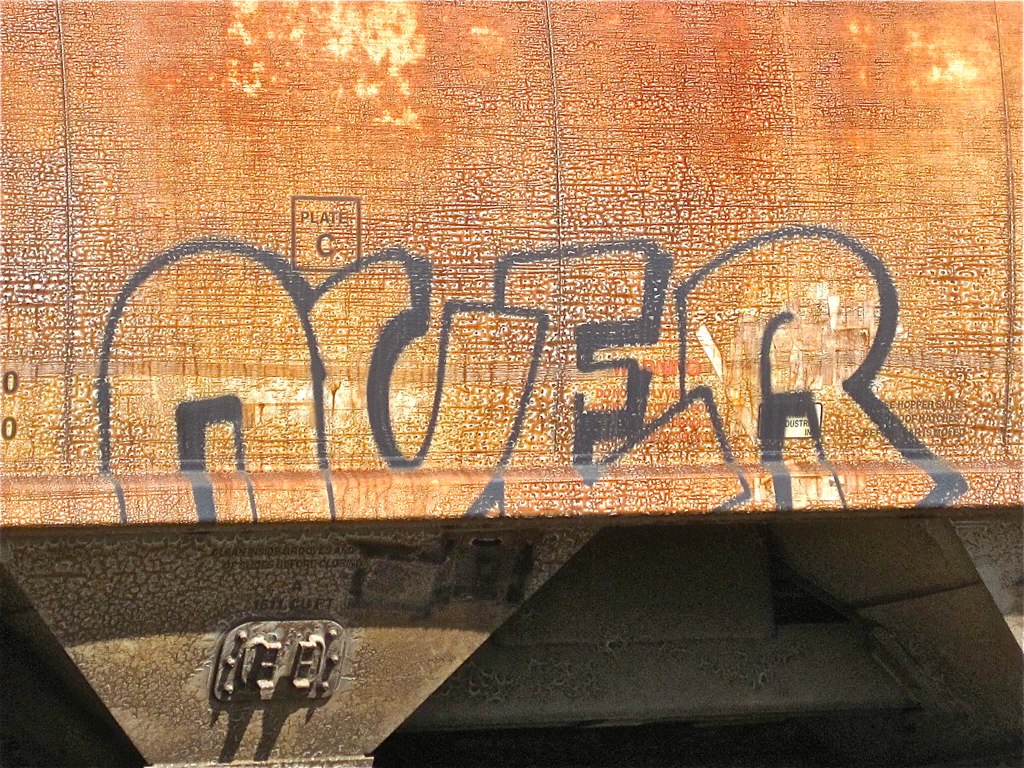This daytime outdoor photograph captures a close-up of a severely rusted railway freight car. The corroded metal, presenting a mix of orange and grimy red hues, serves as the backdrop for black outlined bubble graffiti spelling out "A-C-E-R," with the letters not filled in, allowing the rusted metal to show through. Above the graffiti is a square label with the text "Plate C." On the left side of the frame, a triangular metal bolt extends downward, possibly connecting to a wheel. There are also two zeros visible near this attachment point, suggesting some form of rail car identification.